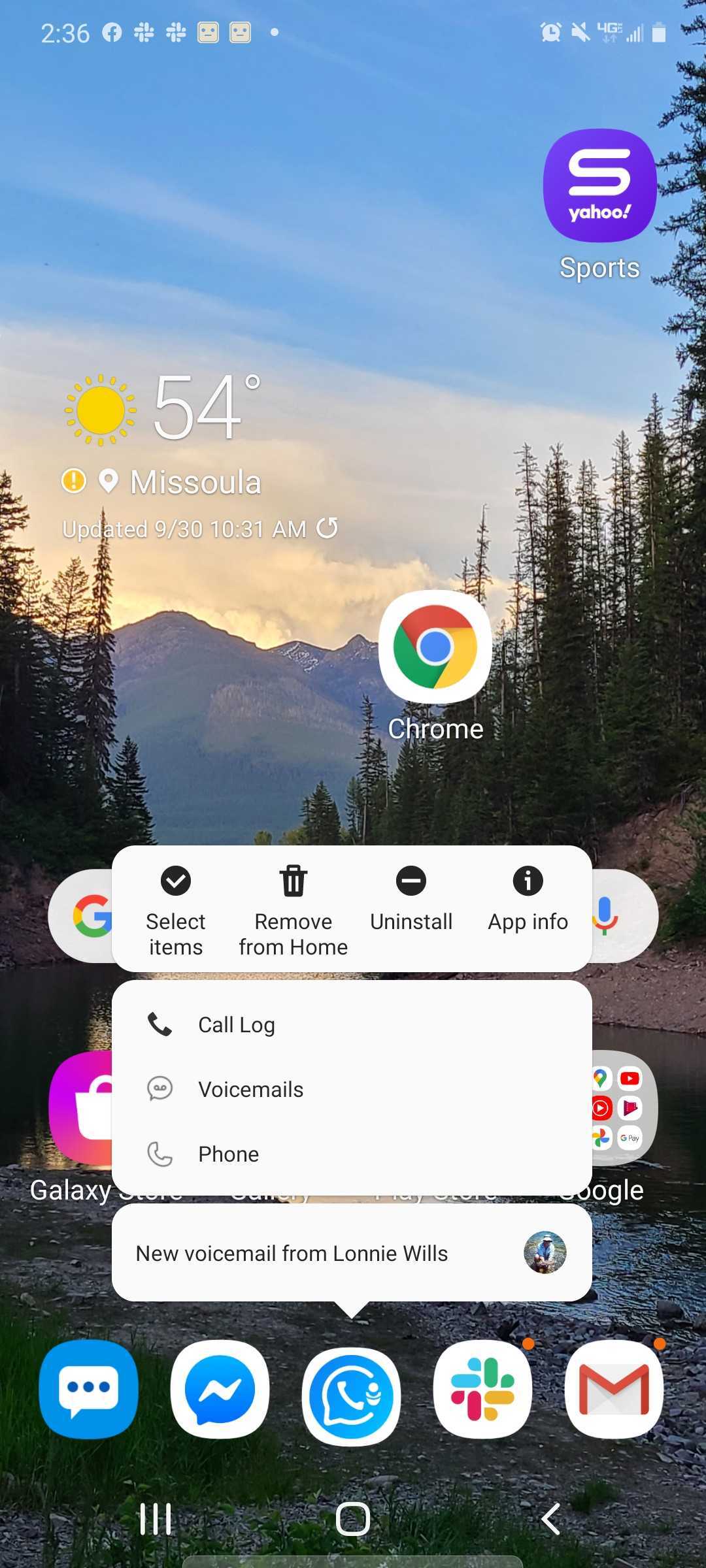A captivating wallpaper adorns a Mozilla phone, showcasing a serene, picturesque nature scene. The image features a gently winding river flanked by tall fir trees and tranquil mountains in the background, capped with clouds that hint at an approaching sunset. The calming natural scene begins to transition into dusk. Centered on this beautiful landscape is a floating Chrome app icon. Below the icon, a dialog box has appeared, displaying options with a checkmark for selecting items, a trash can for removing the app from the home screen, uninstall, and app information. Below the dialog box is a call log featuring a phone emoji, a voicemail box, and a phone icon. Additionally, the home screen features icons for the Galaxy Store and various Google apps, including Google Maps and YouTube. Further down are buttons for messaging, a comment function, and Gmail, indicating unread messages with notification dots beside them.